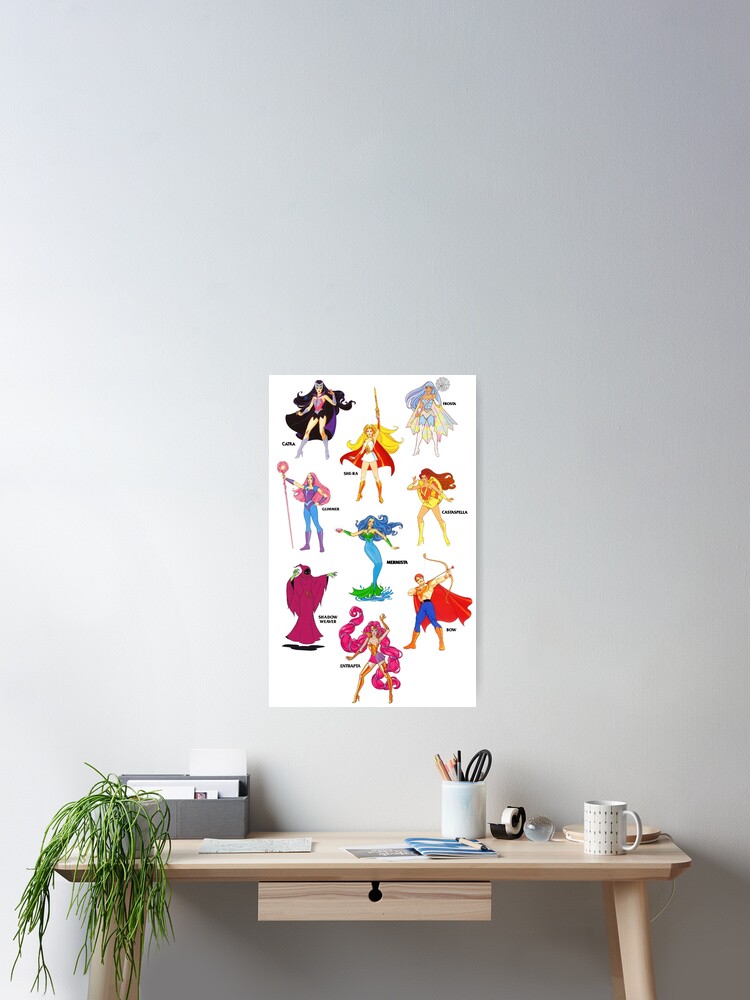The image depicts a vibrant poster featuring nine distinct characters from "She-Ra: Princess of Power," prominently displayed on a light gray wall. Each character is portrayed with vivid details and unique styles against a white background. Central among them is a character with long, wavy blue hair, dressed in a slim blue pant and green top ensemble.

To the left on the poster stands a superhero in a black cape, short mini skirt, and long gray boots, while a character with a red cape, long yellow hair, and a white short skirt brandishes a raised sword nearby. Another superhero, donning long blue pants, a corset-like top, and purple boots, holds a large stick with a circular ornament. 

The poster also features a mermaid-like figure with a blue and green tail and blue hair, a heroine in a yellow skirt and long yellow boots with brown hair, and a character with flowing, long pink hair, wearing a brown corset and thigh-high brown boots. Additionally, there's an ambiguously gendered ghostly figure and a male character equipped with a red cape, blue pants, brown boots, and a bow and arrow.

Below the poster, a light brown wooden table is neatly arranged. On its left side, there is a vibrant green plant with long leaves. Towards the right, a slender white reading lamp stands next to a white cup. Additional items on the table include stationary supplies, a pen stand, a tape holder, and a collection of books and papers, all contributing to a well-organized home decor setup.